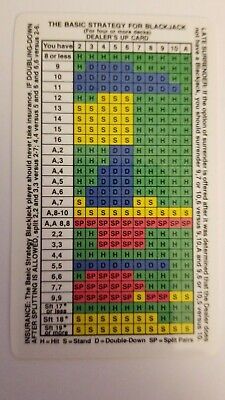This image captures a detailed blackjack strategy chart, prominently titled "The Basic Strategy for Blackjack" in black text at the top. The chart, which appears to be a white card with numerous small letters and numbers, is divided into approximately 20 rows and 12 columns. The first column, labeled "You Have," lists potential initial hand totals ranging from 8 or less up to various combinations of Ace and numbered cards. Horizontally, it extends from 2 through 10 and Ace, representing the dealer's visible card.

Each cell within the grid is color-coded—green for "Hit" (H), yellow for "Stand" (S), blue for "Double Down" (D), and red for "Split" (SP). These colors and corresponding letters offer clear, quick-reference actions for each possible hand scenario. Additional small black text framing the chart spells out what each color and letter signify. Despite the clarity of the color-coding, the smaller text details and explanatory notes around the edges are somewhat difficult to read due to their size. The overall effect is a highly structured, multicolored guide designed to assist players in making optimal decisions in every situation encountered during a game of blackjack.